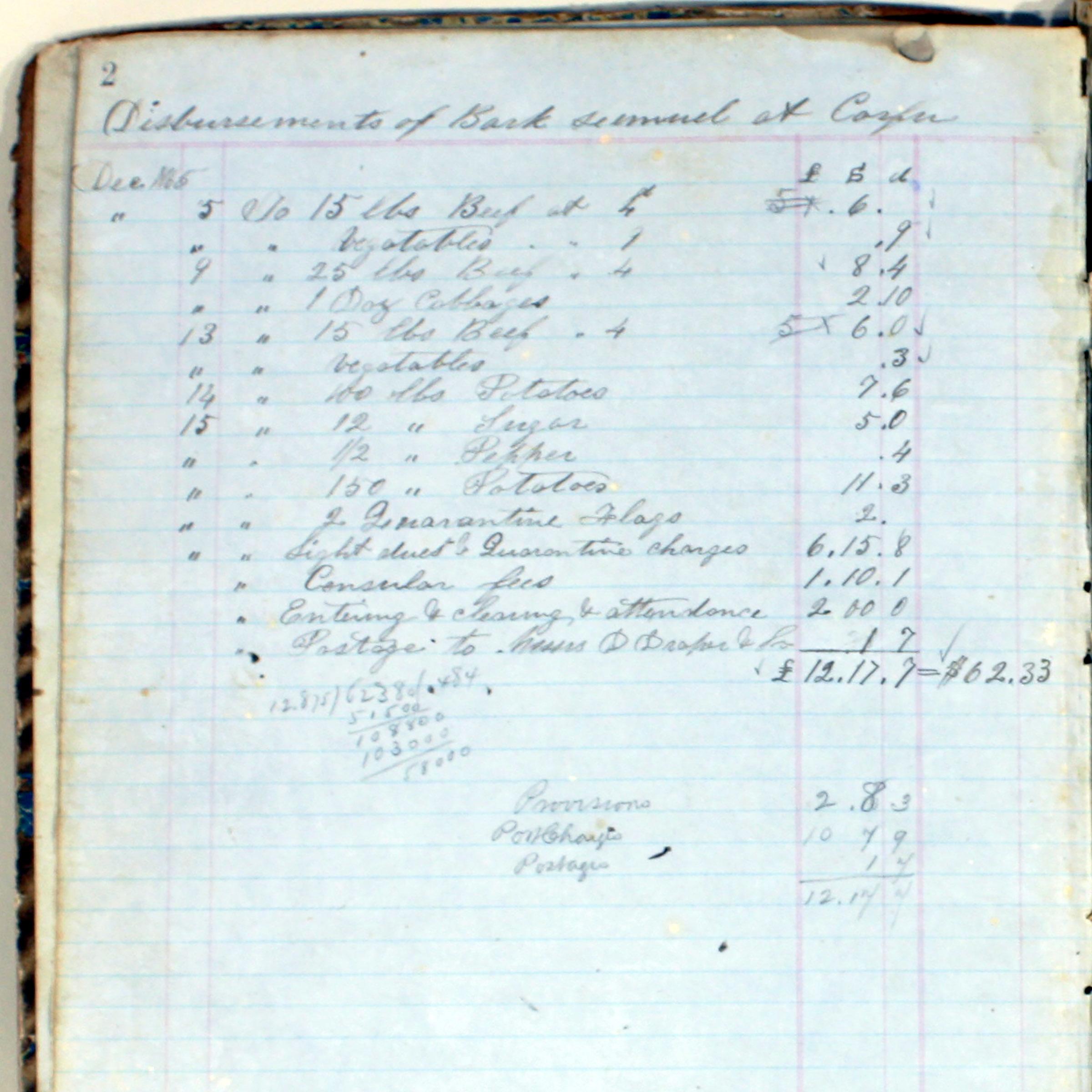The image depicts an aged and slightly worn page from a lined writing exercise book, possibly used for historical or accounting purposes. The paper, showing both blue horizontal and pink vertical lines, features elegant cursive handwriting, likely written in pencil. Prominently titled "Disbursement of Banks" in cursive, the document appears to be an accounts payable register from December, detailing various expenses. The left column lists several items or vendors, while the right column shows amounts, primarily in Euros, including a total of 12.17 Euros. Additional calculations and doodles are visible in the margins. Notable details include the page number "2" in the top left corner and a tick mark amidst the listed amounts. The conversion of the total amount to dollars (62.33) is also noted at the bottom.